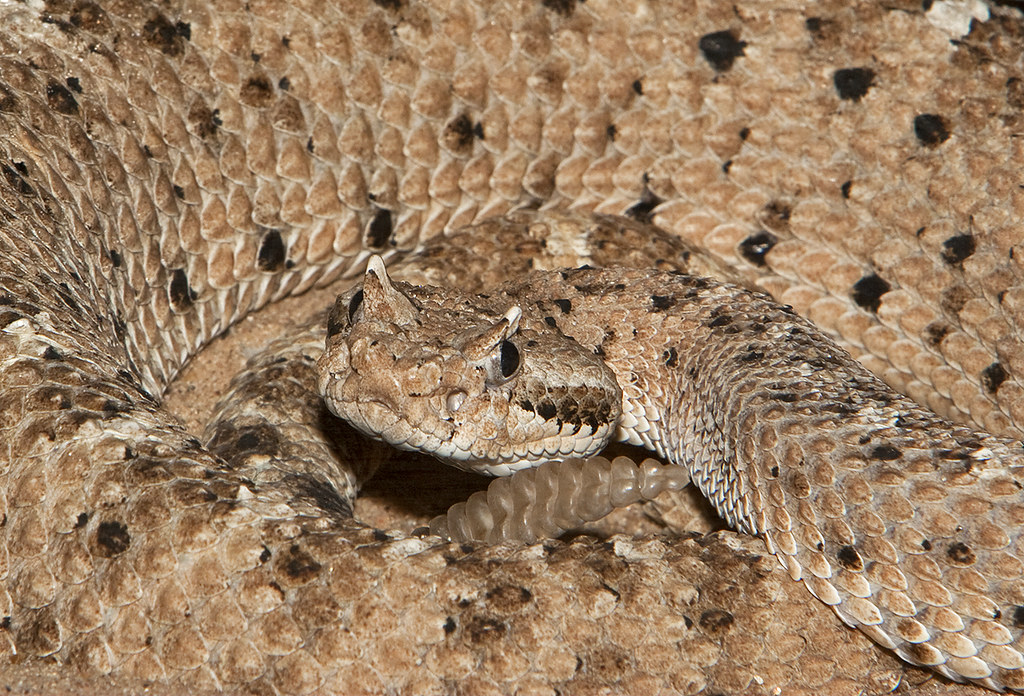This close-up photograph captures a coiled rattlesnake, with its head prominently centered in the middle of the image. The snake's sand-colored scales, flecked with brown and black, provide it with excellent camouflage, blending seamlessly with its surroundings to the point where the body could be mistaken for the sandy ground. The snake's head, featuring prominent dark eyes with black pupils, gazes straight at the camera, giving an impression of relaxed caution. The rattle of its tail, a clear tan and light brown, peeks out from beneath its coiled body, adding to the snake's distinctive appearance. The bright, detailed image reveals a creature at rest, its closed mouth suggesting it is not in an aggressive state. Overall, the intricately coiled body and the snake's textured pattern evoke the illusion of a braided rug or a cat bed at first glance, but closer inspection reveals the rattlesnake's true nature.